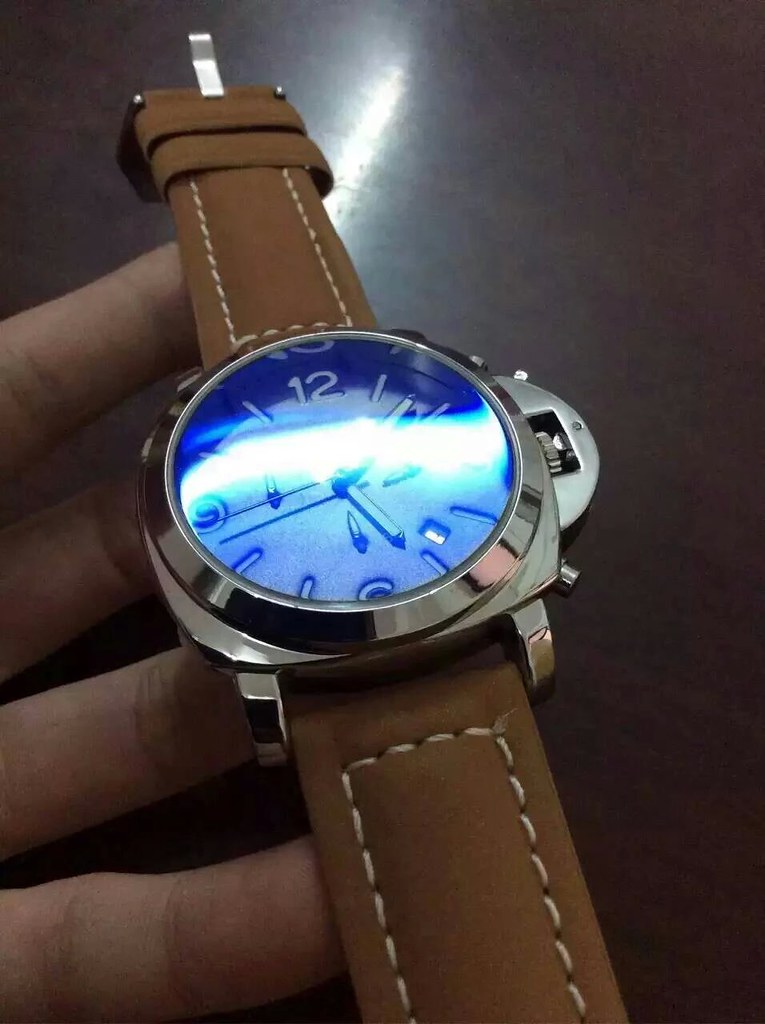In the image, a hand—presumably the left one given the absence of the thumb—is holding a wristwatch across its four fingers. The watch features a brown leather band with light-colored stitching along the edges, giving it a slightly velvety texture. The band fastens with a clasp, though the specific type isn't clear. The watch itself has a substantial, silver or steel bezel, accented by buttons on the right side, and a protected stem. Its face is blue, displaying the time around 5:08. Notably, the analog watch shows only the numbers 12, 3, 6, and 9, with white indices filling the gaps. The second hand sweeps smoothly across the blue background. In the right section of the watch face, a small date window with a white background and black numerals adds to the detailed design. The background of the image reveals a sleek, washable silver table, typical of kitchen settings. Harsh fluorescent lighting creates a bit of glare, emphasizing the metallic elements of the watch and table.